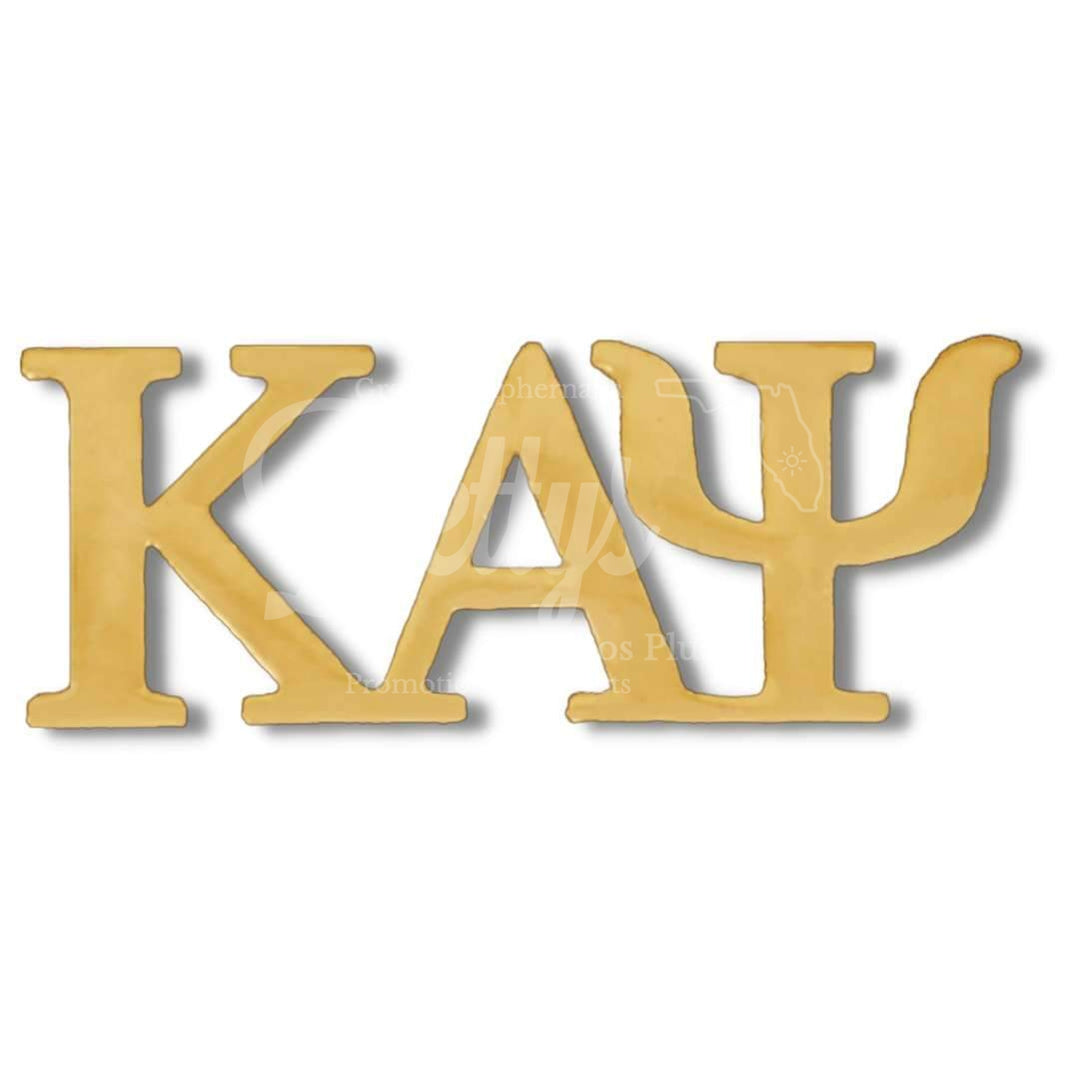The image features a simple, yet intricately designed typography. Set against a white background, three large, capitalized letters in a gold color spell out "KAY." The letters are serif and appear to be connected at the bottom, forming a continuous line that stretches from the base of the K, through the A, and finally to the unusual depiction of the Y. The Y in particular stands out with wavy, arm-like extensions that curve upward and outward on both sides, resembling a large, stylized Y or possibly even an intricate I. The text has a hand-drawn, black-bordered relief effect, giving it a shadowy, suspended appearance. There is also a very transparent watermark over the letters, so faint that it is difficult to make out. This creative arrangement and styling of the letters present a unique and elaborate representation of the name "KAY."